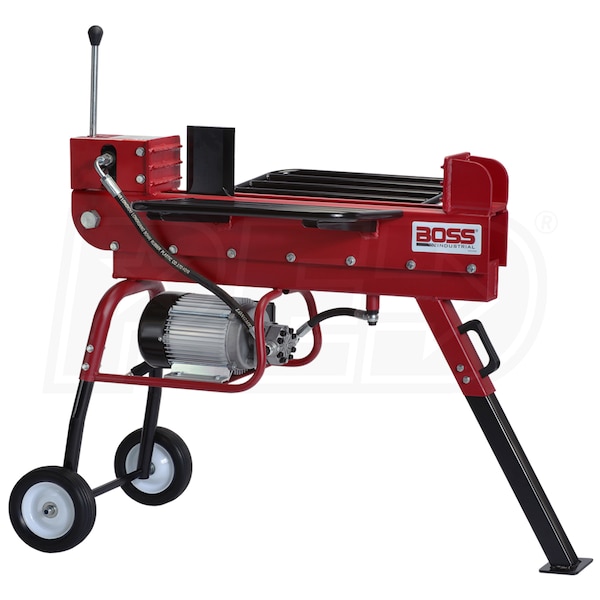The photograph displays a red piece of power equipment resembling a portable grill on a white background. The top section features a red structure with foldable metallic boards that angle inwards when propped up. Prominently, a white label with red "BOSS" lettering and the word “Industrial” is affixed to the right side of the device. Below this red top component is a compact, silver electric motor with a black cap, connected via two hoses to the main structure. Supporting the equipment are two black, wagon-like wheels on the left, and a single adjustable kickstand on the right. A red post alongside a handle on the left side suggests mobility and stability, adding to the impression of multi-terrain usability.